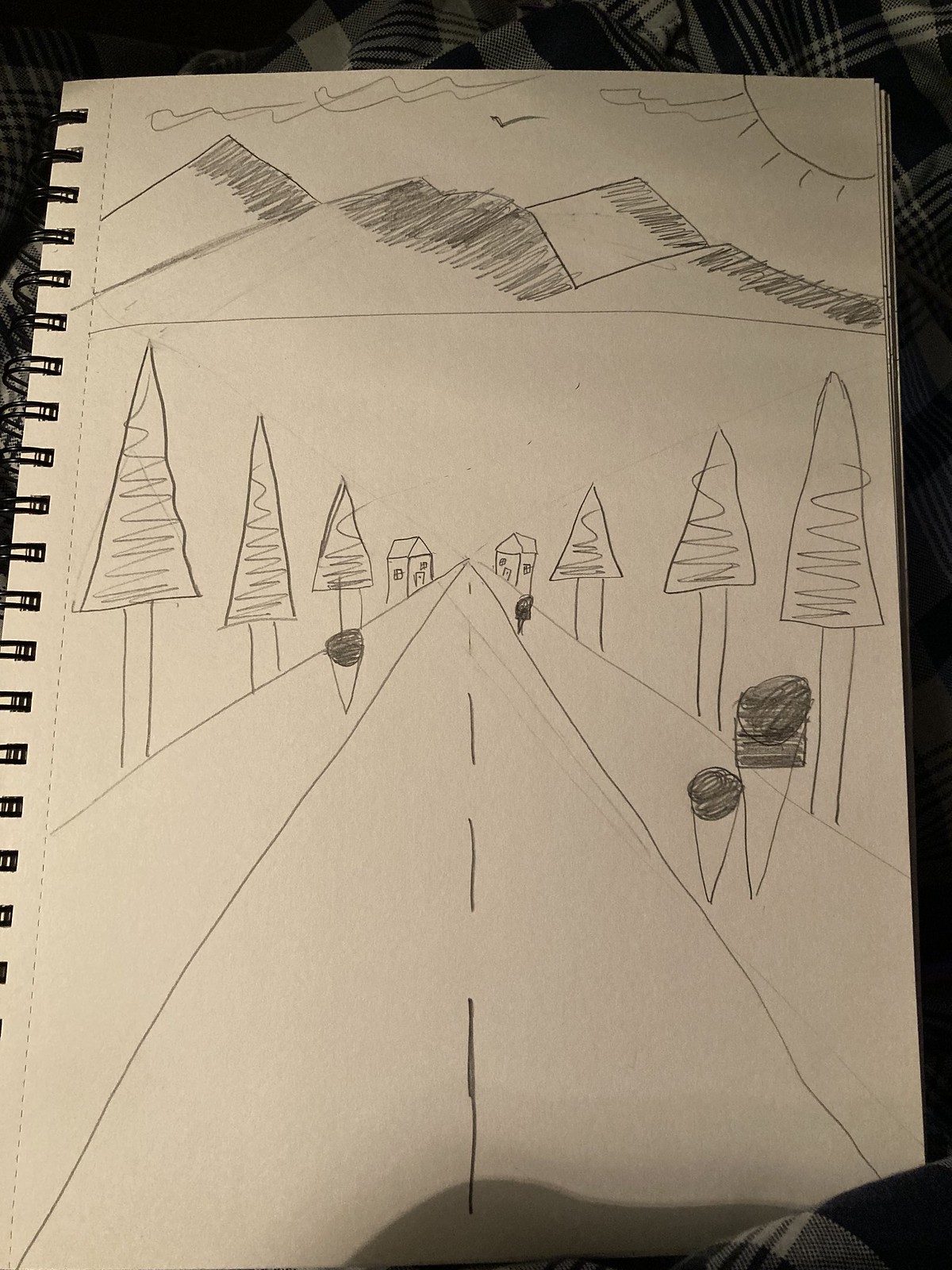This detailed black pen drawing on off-white sketch paper, bound in a spiral notebook with the spiral on the left-hand side, captures a serene landscape scene. The top of the page features squiggly lines suggesting clouds, with a V-shaped line representing a bird gracefully flying above. In the upper right-hand corner, a sun radiates light with small lines extending outwards, while triangular mountains with shaded peaks stretch across the horizon.

Dominating the composition is a long road extending straight from the bottom of the page into the distance, marked by a dotted centerline. Rows of trees, characterized by long, skinny trunks and triangular canopies filled with intricate squiggly details, line both sides of the road. Nestled along the road are two quaint houses, placed symmetrically near the end of the street, one on each side, creating a comforting sense of symmetry and balance.

On the bottom right of the sketch, there appears to be two ice cream cones, whimsically placed on the side of the road, and a piece of flannel clothing. The overall effect is a charming, detailed illustration, offering a glimpse into an artist's tranquil depiction of a picturesque landscape.